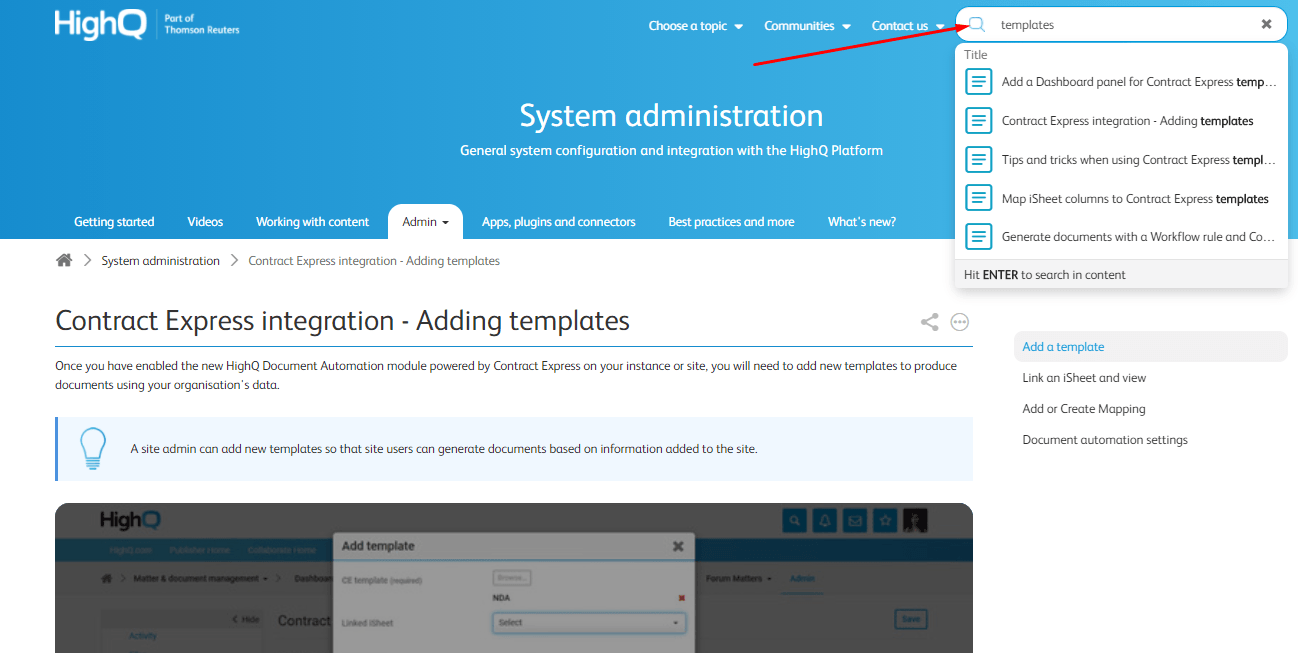The image depicts a website interface with a blue header at the top. On the top-left corner of the header, the logo "HiQ" is displayed in white text. In the center of the blue header, the words "System Administration" are prominently shown.

The top navigation bar, also within the blue header, includes clickable options in white text: "Choose Topic," "Communities," and "Contact Us," each accompanied by a downward-pointing white arrow. To the right of the "Contact Us" option, there is a white search bar with a blue magnifying glass icon. The search bar contains some text, possibly "templates," but it's too blurry to decipher clearly. 

Below the blue header, several sections are listed: "Getting Started," "Videos," "Working with Content," "Admin," "Apps, Plug-ins, and Connectors," "Best Practices and More," and "What's New." The "Admin" section is currently selected, and the content underneath is specifically about this category. The white area below the header presents detailed information on "Contract Express Integration" and "Adding Templates." 

Accompanying this content is a small gray box featuring a blue light bulb icon. The text in this section is in black font, though it is somewhat blurry and difficult to read. 

Beneath this, there is another gray box which appears to be a snapshot from a different webpage. It includes the phrase "Add Template," but this text too is hard to read due to blurriness.